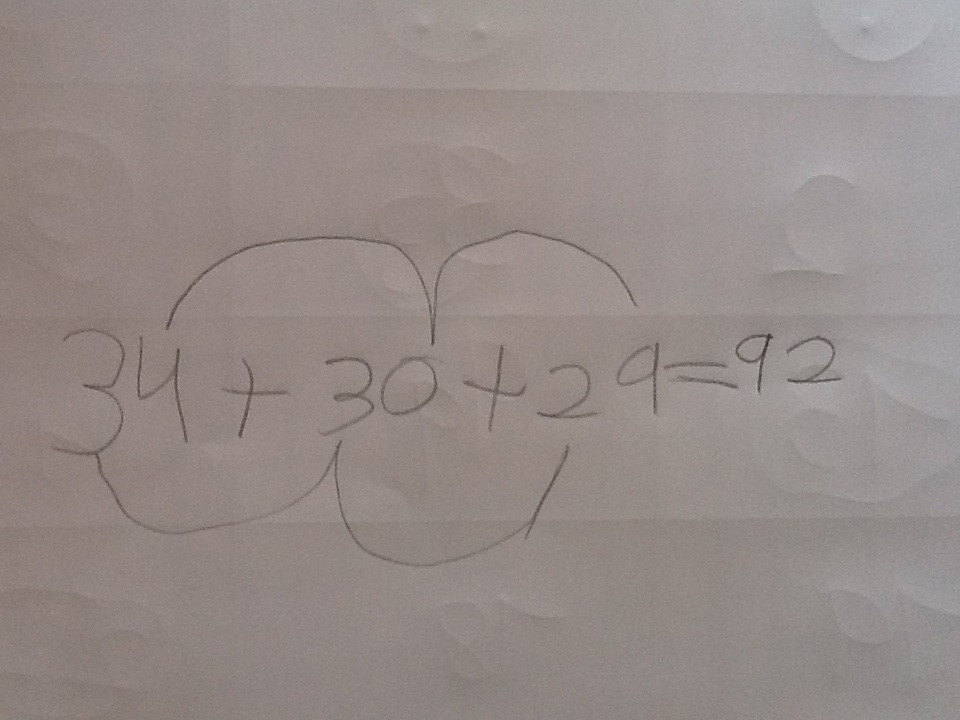This highly detailed, close-up image captures a math problem meticulously written on a light gray piece of paper. The problem spans most of the horizontal space in the middle of the page, flanked by empty margins at the top and bottom. Through the paper, one can faintly discern outlines of reversed numbers from the opposite side, likely due to the pressure from the pencil writing. Particularly, you can make out what appears to be a reversed 70, 78, 2, 33, and 73, among others, suggesting approximately seven or eight distinct numeric impressions.

In the foreground, the math problem prominently displays the equation "34 + 30 + 29 = 92." Above this equation, two squiggly lines offer guidance on how to perform the calculation, possibly indicating intermediary steps or the overall thought process behind arriving at the correct sum. The handwriting suggests that a child might have written the problem, adding a layer of innocence and learning to the scene.